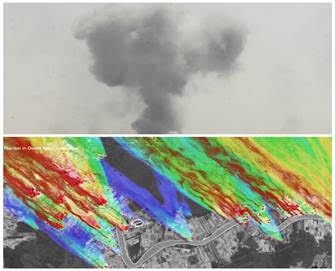The image is a composite divided into two distinct halves. The top half features a large plume of smoke resembling the iconic mushroom cloud from an atomic bomb, set against a smoky gray background. The smoke thickens as it rises, composed of various shades of gray. Below, the picture transforms into a vibrant, abstract aerial view. This segment is marked by streaks of red, blue, green, turquoise, yellow, and indigo slanting from the top left to the bottom right. There are black and gray scribblings near the bottom of this portion, contributing to the chaotic yet artistic appearance. Amidst the colorful patterns, there can be hints of a road and possibly some obscured terrain like a city or pasture, evoking images of lava flow over a landscape.